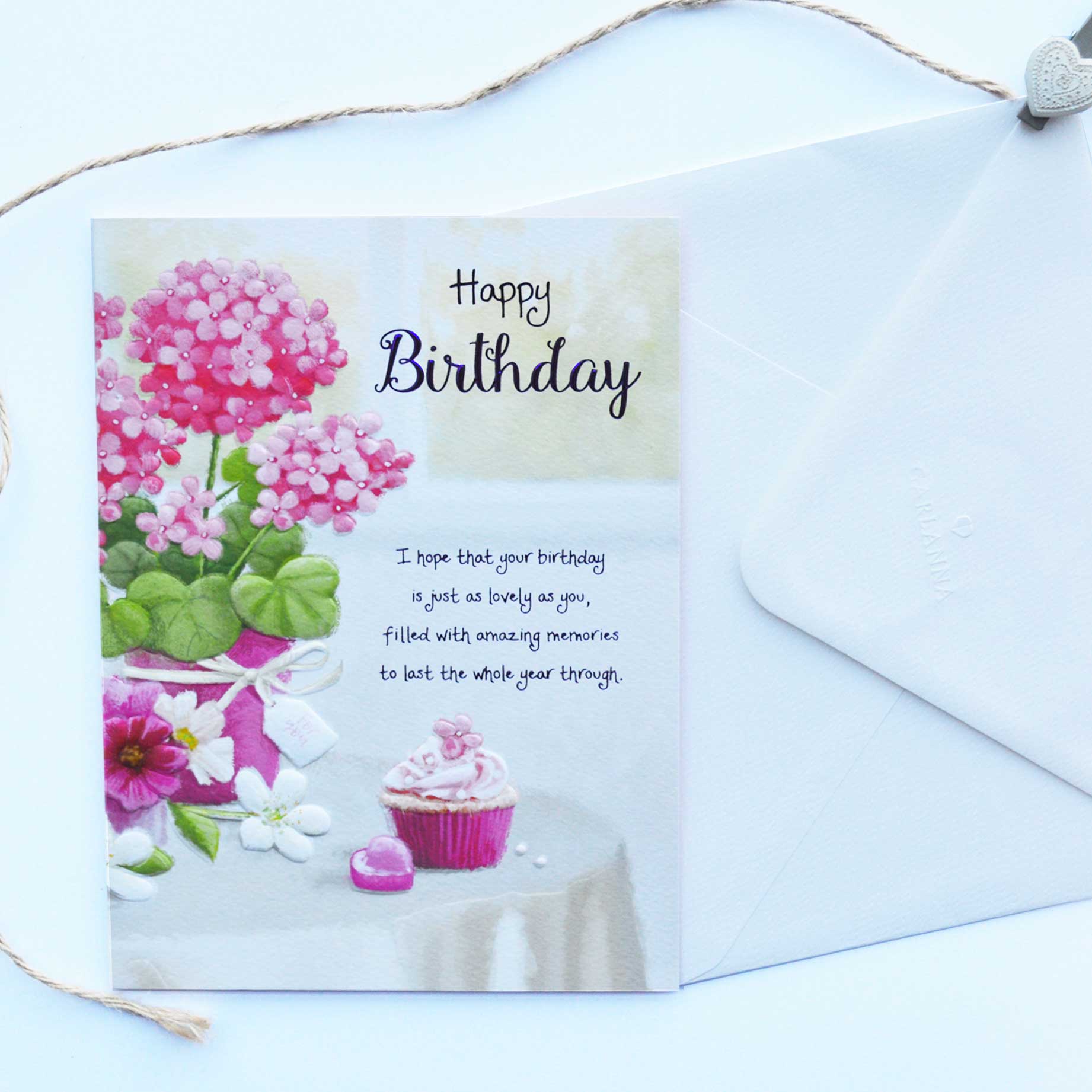The image features a vividly detailed birthday card partially slipped into a white envelope, all placed on a white table. The card, predominantly light blue and approximately seven inches wide, occupies the left section, while the envelope sits to the right. Adorning the card’s pale blue background, a charming illustration dominates with a pink flower pot housing pink blossoms with large green leaves, tied delicately with a white butterfly. Surrounding the pot, there are larger purple flowers, white flowers, and a heart-shaped pink accent. Next to this vibrant array is a cupcake with white frosting in a pink cup. The card contains an ornate greeting in dark, elegant typeface that reads: "Happy Birthday," with a heartfelt message below in smaller, stylish letters: "I hope that your birthday is just as lovely as you, filled with amazing memories to last the whole year through." A pink piece of string meanders through the composition, suggesting a personal and tender touch to the scene.